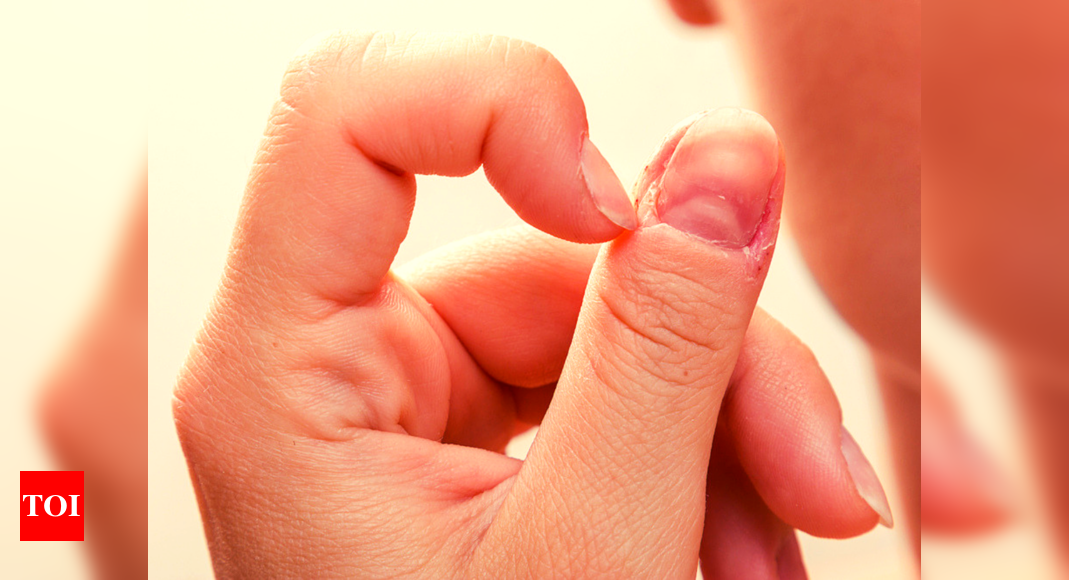The photograph features a close-up of a light-skinned hand in front of a pale cream background, with part of the cheek and lower ear also visible. The hand is positioned beside the face, with the main focus on the thumb and index finger. The index finger is touching the thumb, seemingly picking at the cuticle, which appears ragged and worn, with evident signs of irritation and raw edges. The fingernails are unmanicured, displaying torn cuticles and a generally raggedy appearance. Behind the thumb, the middle and ring fingers are partially visible. In the bottom left-hand corner of the image, there's a logo in a red square with white serif letters spelling "T O I."